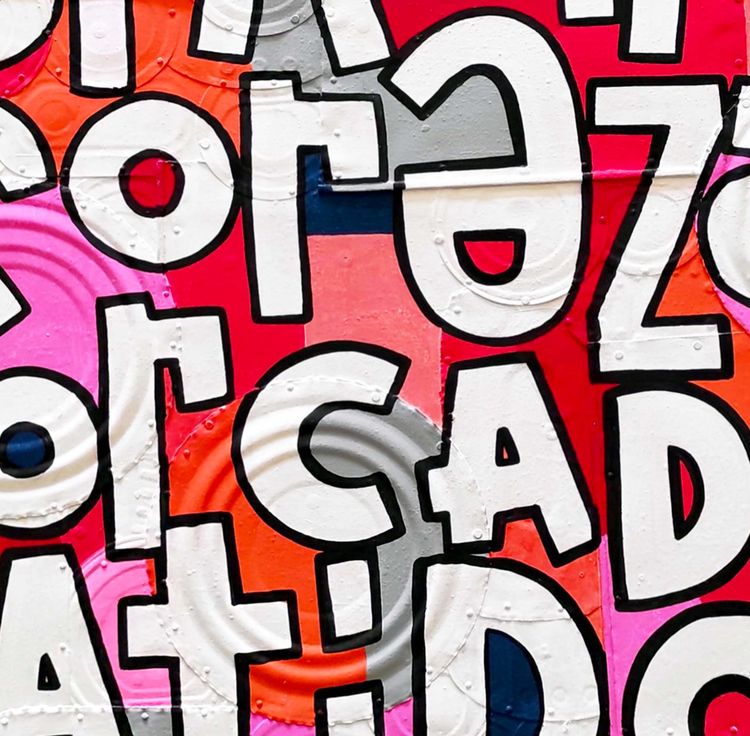This image is a close-up, zoomed-in photograph capturing a section of a wall or possibly the side of a truck, heavily adorned with graffiti. The image prominently features large, white letters outlined in thick black strokes, arranged randomly and in various orientations—some are right side up, some upside down, and others might even be backwards. The visible letters include O, R, E, Z, R, C, A, D, T, and I, although no complete words can be deciphered due to the cropped nature of the image. The background is a vibrant mix of colors, including shades of red, pink, peach, and orange, creating a chaotic but visually intriguing canvas. The letters are sprawled across the top, middle, and bottom rows, though the composition makes it difficult to discern any specific pattern or language. Overall, the colorful backdrop and abstract arrangement of letters give the scene a dynamic, layered aesthetic.